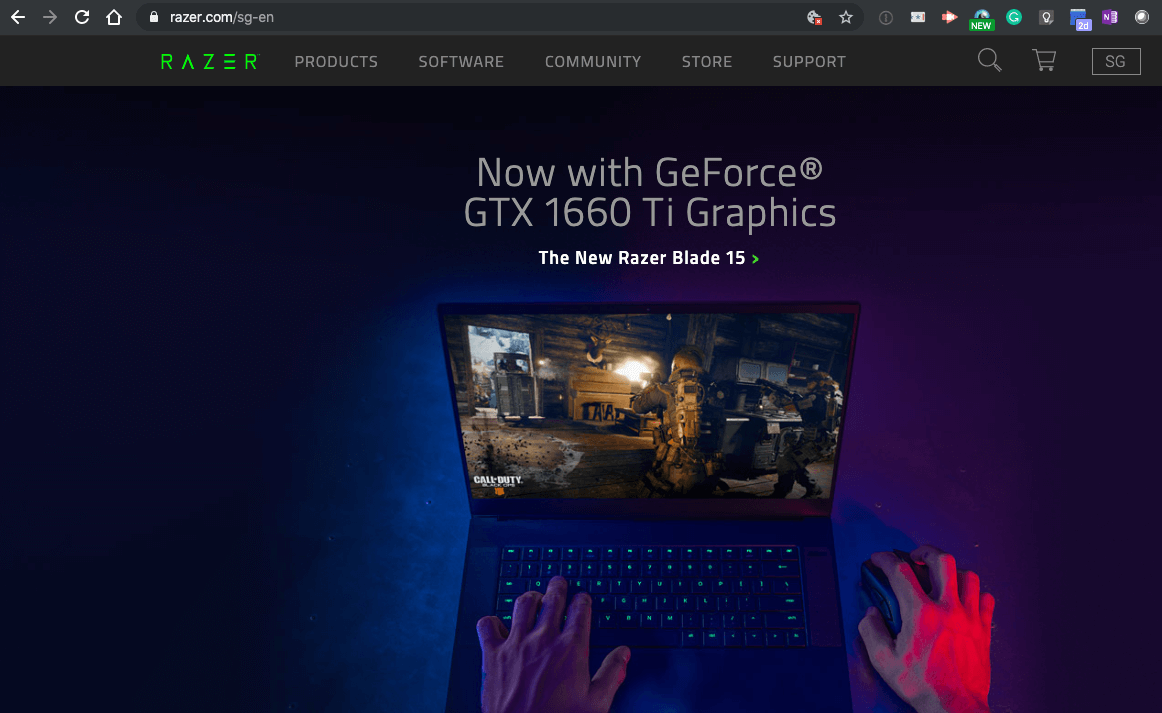This screenshot captures the intricate details of a website's homepage. At the very top, there is a medium gray header featuring several navigation icons: a white leftward arrow on the left, followed by a light gray rightward arrow, a white refresh icon, and a white home icon. Adjacent to these icons is a dark gray URL bar, starting with a white lock icon on the left and continuing with the text "razor.com" in white, followed by medium gray text "/SG-EN". To the far right of the URL bar, there is a white globe icon with a red box on its bottom right corner, and a white star icon. Outside this URL bar setup, several multicolored icons are aligned to the right.

Beneath the header lies the homepage's primary content, starting with a very dark gray navigation bar. To the left of this bar, green stylized text reads "RAZOR," with unique design elements: the horizontal line in the 'A' and the vertical line in the 'E' are missing. Toward the right of this logo, light gray uppercase text lists the site’s main sections: "PRODUCTS", "SOFTWARE", "COMMUNITY", "STORE", and "SUPPORT". Following a gap, there are three more icons on the far right: a light gray magnifying glass (search), a shopping cart, and a rectangular outline with the letters "SG" inside.

The body of the webpage showcases a central image featuring a laptop. The laptop’s keyboard keys are illuminated in green, and the screen displays a shooter video game with the title "CALL OF DUTY" in white text, amidst a gray-brown tinged scene in the bottom left. A hand is positioned on the left side of the keypad, and another hand, illuminated by pink light, is holding a mouse to the right of the laptop. The laptop screen also exhibits an illuminated blue splotch, adding a distinctive visual contrast.